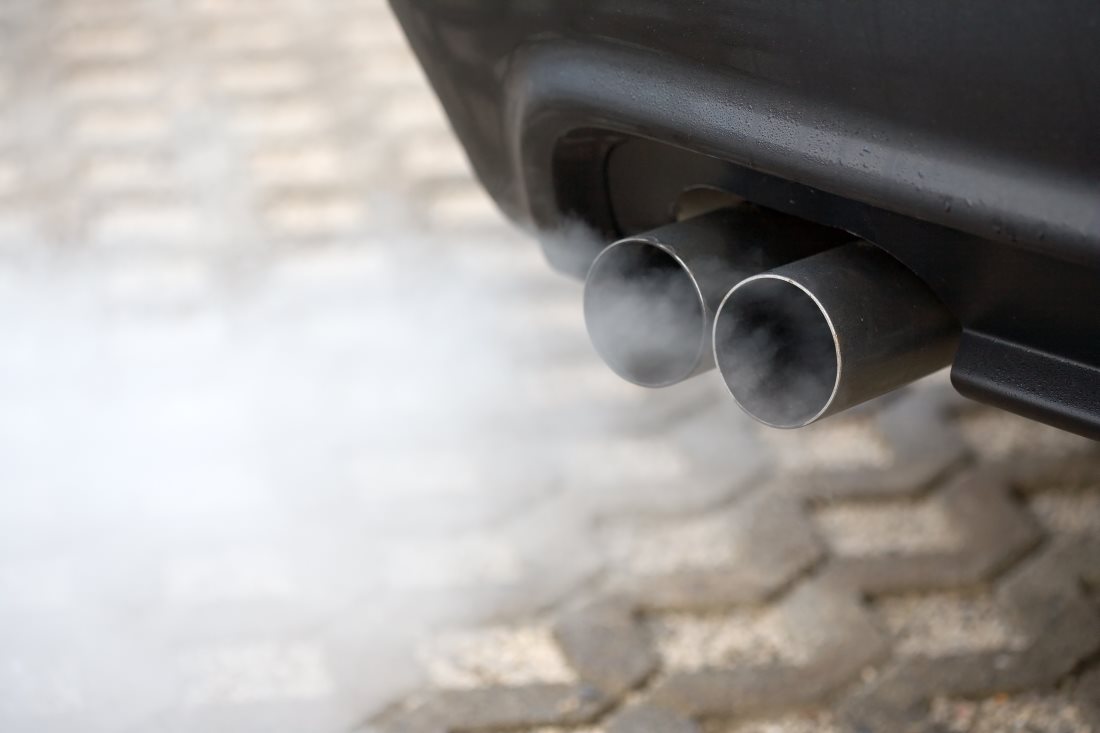The image is a detailed close-up of a car's dual exhaust pipes with significant emphasis on the surrounding elements. The photograph captures the bottom left-hand side of the car, focusing on the silver exhaust pipes which are positioned side-by-side, emitting billowing whitish-gray smoke. The car's exterior appears to be black with a slight sheen, suggesting it might be wet, although the detail is somewhat blurry. The visible fender in the upper right corner of the image is gray. Below the exhaust, the ground features a distinct v-shaped tread pattern, resembling small beige-brown mountains against a yellowish background. The tread extends from the lower right to the upper left corner of the image, filling the space not occupied by the car.